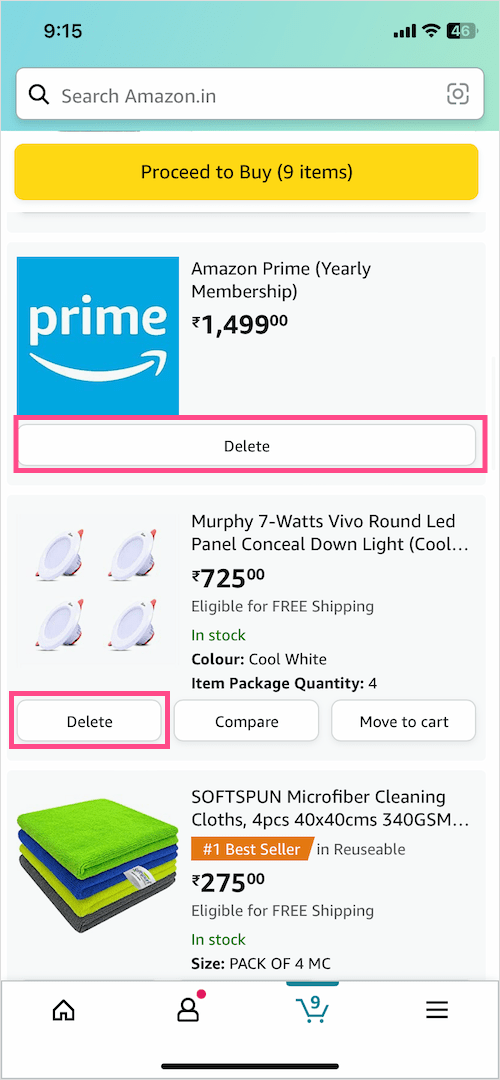This screenshot captures an Amazon.in page displayed on a mobile phone. At the top, a status bar with a blue background shows the current time as 9:15 in black text on the upper left. In the upper right, indicators for reception strength, a Wi-Fi icon, and a battery icon displaying 46% charge are visible.

Below the status bar, a search bar with a magnifying glass icon features the placeholder text, "Search Amazon.in." Beneath the search bar, a prominent yellow button with the inscription "Proceed to Buy" in black text is shown, indicating that there are 9 items ready for purchase.

The first item in the listing is an Amazon Prime yearly membership priced at ₹1,499. This entry sports the word "Prime" in white text accompanied by the Amazon smile logo on a darker blue background. Additionally, a magenta-outlined "Delete" option is available beneath this listing.

Following the Prime membership, the next product listed is the "Murphy 7 Watts Vivo Round LED Panel Concealed Down Light" priced at ₹725. The final visible item in the screenshot is a set of "Soft Spun Microfiber Cleaning Cloths" priced at ₹275 for four pieces.